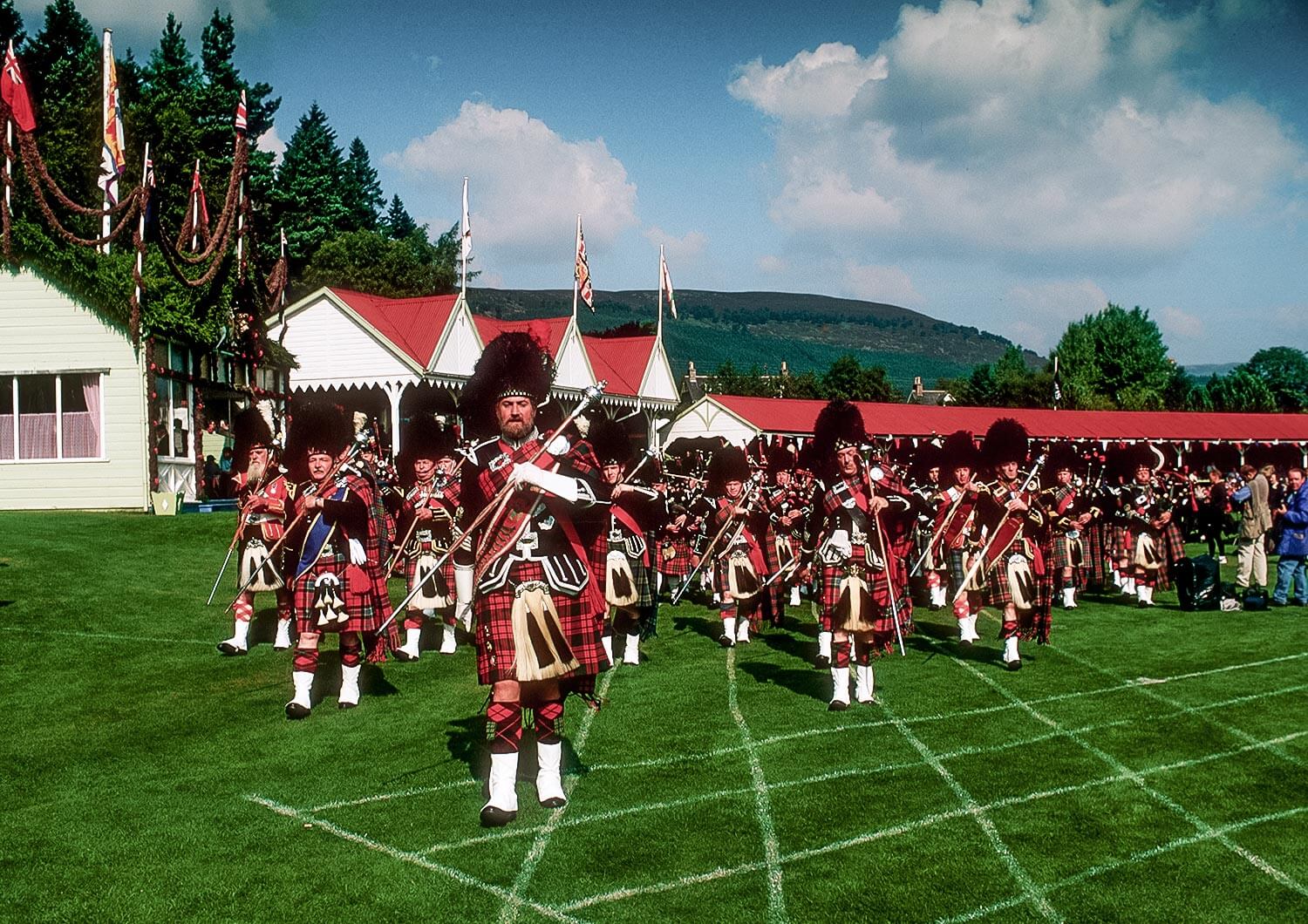The image depicts a Scottish marching band performing on a well-manicured green lawn, which features a grid of white lines forming rectangles and squares in the lower right corner. The band is led by a man positioned just left of center, identifiable by his tall black hat and red and black plaid kilt, accented with a tan brush-like sporran at the front waist. He holds a large stick, possibly a baton, in his left hand. 

Rows of band members dressed similarly in red and black plaid uniforms—with knee-high white socks and dark-colored hats—follow behind him. Each musician carries a thin silver pole topped with a shiny, doorknob-like bulb. The performers are uniformly marching in formation.

To the right of the band, spectators observe the parade. The background features various buildings: a white building with a green roof and decorative elements, a larger structure with three pointed roof sections, and an elongated building stretching off the right side of the image. Behind these structures, evergreen trees are visible under a blue sky dotted with white clouds. To the left of the image, a small hillside slopes upwards, adding to the scenic backdrop.